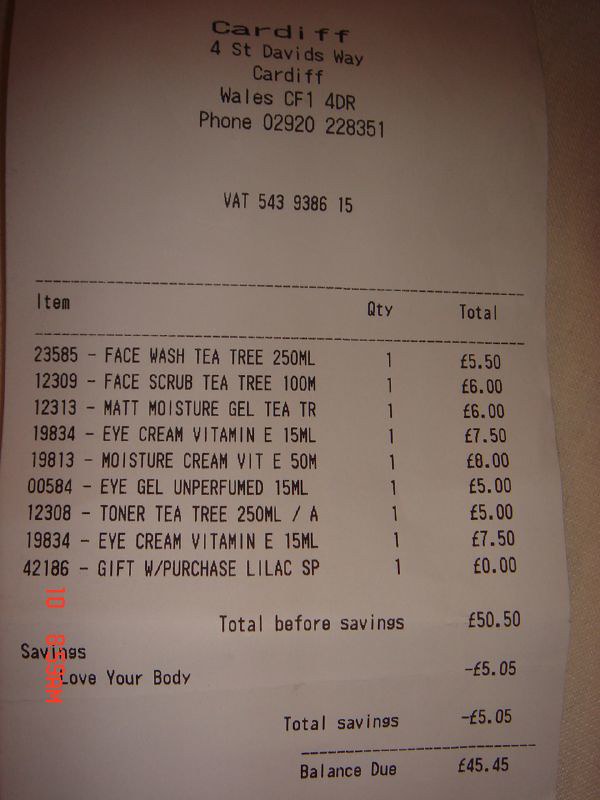This image captures a detailed receipt from Cardiff, prominently displaying the address at 4 ST David's Way, Cardiff, Wales CF1 4DR, alongside a phone number at the top. Below this, VAT number 543-9386-15 is listed. The receipt is printed in stark black text on a white background. It features a dotted line separating the header from the itemized purchase details, which include quantities and totals for each product. The items purchased are: Face Wash Tea Tree (250 ml), Face Scrub Tea Tree (100 ml), Matte Moisture Gel Tea (TR), Eye Cream Vitamin E (15 ml), Moisture Cream Vitamin E (50 ml), Eye Gel Unperfumed (15 ml), Toner Tea Tree (250 ml), Eye Cream Vitamin E (15 ml), and a Gift with Purchase (Lilac SP). The financial summary at the bottom indicates a total before savings of £50.50, a discount of £5.05, resulting in a balance due of £45.45. The receipt also includes a note, "savings, love your body," emphasizing the discount.